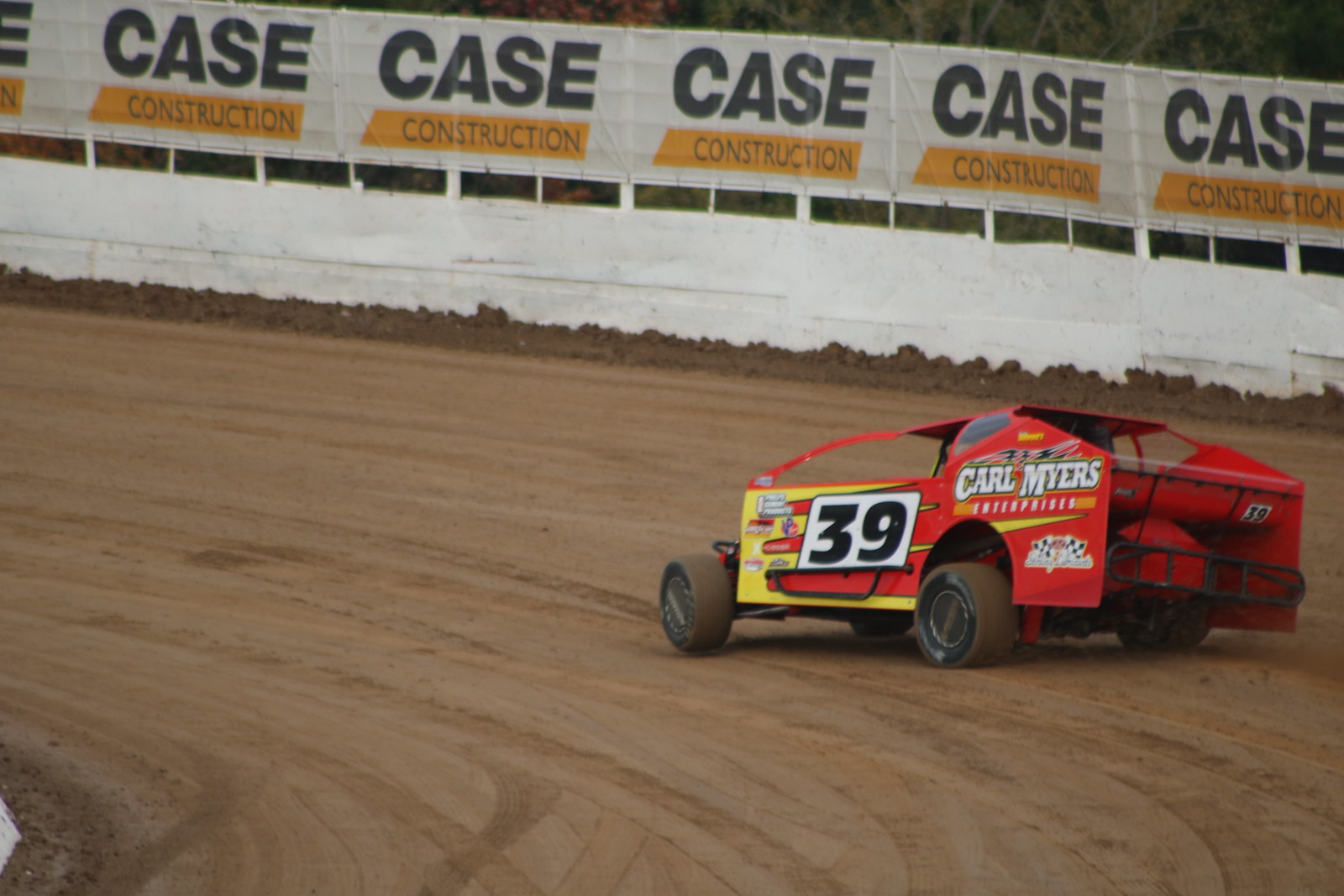This image captures an action shot of a red amateur race car sliding around a muddy, brown dirt track. The car, marked with the number 39 in prominent white digits, features a steel frame and the name "Carl Myers Enterprises" emblazoned on the side, along with yellow flame decals. It rides on four black, smooth tires. The action is taking place on a dirt racetrack bordered by a white fence adorned with repeating banners advertising "CASE Construction" in large blue and thin black letters against an orange background. In the background, trees can be seen, adding to the outdoor setting of this thrilling scene.